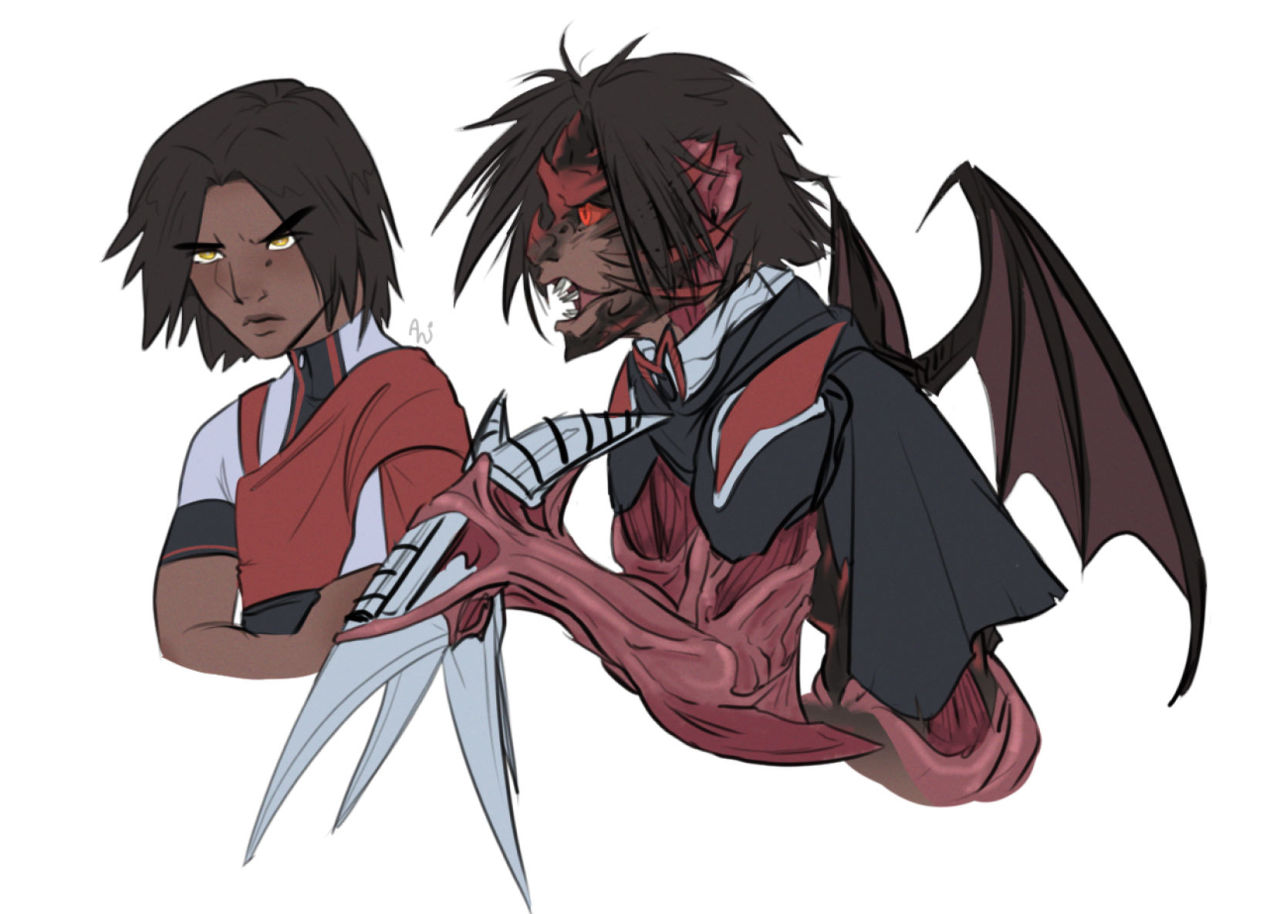This detailed anime-style drawing illustrates a transformative dual depiction of a single character. On the left, a young person with shoulder-length black hair, piercing yellow eyes, and a slight scowl is seen from the waist up. They wear a short-sleeved shirt with red, black, and white stripes, accented by a distinctive red scarf that wraps under their right arm and drapes over their left shoulder. On the right, the same individual appears transformed into a winged creature with disheveled hair and intense red eyes. This menacing form features fangs, a werewolf-like face, and red, muscle-revealing skin, highlighted by a black cape with red spikes and small bat-like wings. The creature's appendages end in sharp, metallic claws, adding to the brooding and fearsome ambiance of the scene.